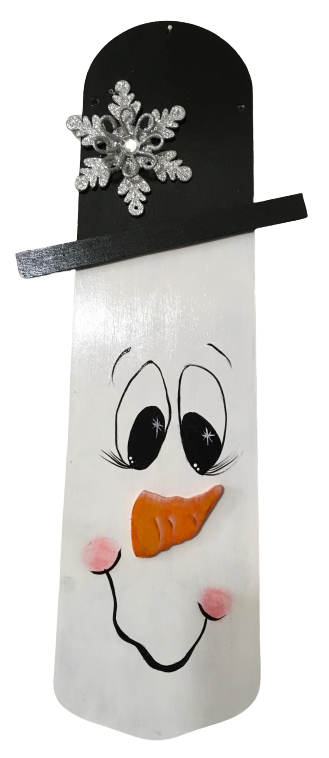The image showcases a craft piece that resembles a snowman's face. The snowman is painted on a flat wooden board with a white background. The board is almost rectangular, with slightly curved ends and a wider bottom side. The top section of the board, painted black, forms a top hat adorned with a gray snowflake. The snowman has cheerful features: black and white eyes with eyelashes and a sparkle, an orange carrot-shaped nose, and a crooked, slightly smiling black mouth with red or pink cheeks. The overall expression of the snowman is happy and festive.